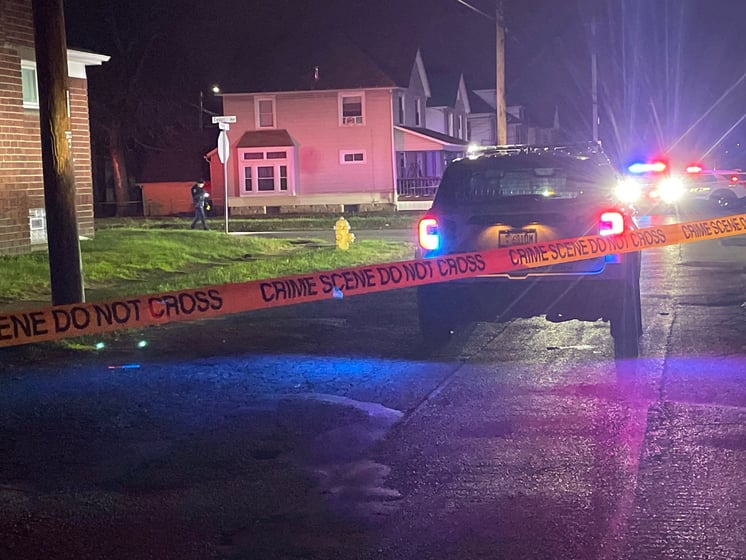In the nighttime scene of a rain-dampened neighborhood, multiple police cars with flashing lights array in various colors—yellow, white, and blue—line the street, their lights creating a blurred, glaring reflection off the wet road. Dominating the scene is a yellow "Crime Scene Do Not Cross" tape with black text that stretches across the street behind a passenger car with its headlights on. To the left, a police officer in a dark uniform, flashlight in hand, appears somewhat blurred as he walks down a side street. Nearby, a two-story pink house stands prominently behind the rows of police cars, while other residential houses, including a red brick one with a green grassy yard, dot the background. The scene is punctuated by urban elements such as a brown electrical pole, a wooden stump likely another pole, a yellow fire hydrant, and a stop sign, highlighting the gravity of the situation in this otherwise quiet residential area.